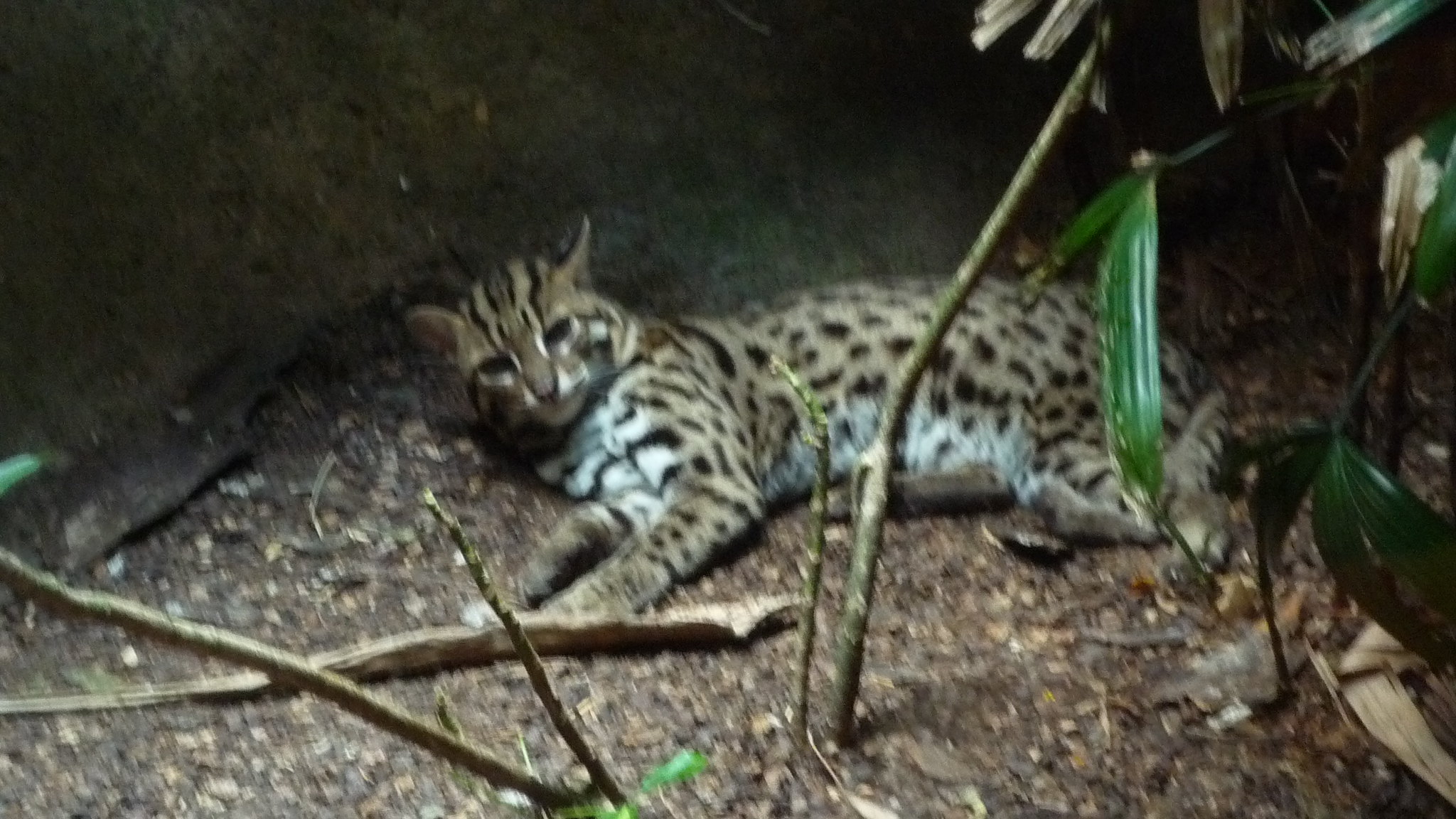This image captures a leopard in its natural habitat, nestled in a small cave-like hiding ground. The leopard, displaying an elegant coat of yellow-brown color adorned with intricate black spots and stripes, is lying on the ground with its head propped up and eyes half-open, giving it an alert yet relaxed demeanor. Its face is framed with striking black stripes, contrasting sharply with the white fur around its mouth, chest, and underbelly, which are also punctuated by black dots. In the foreground, green-leaved plants and scattered debris from surrounding vegetation add to the natural setting. The background features a sloped rock wall, creating a shaded and slightly dark enclosure, possibly hinting at an outdoor environment or a well-crafted zoo habitat. The leopard gazes directly at the camera, its ears and face marked with nuanced dark patterns, exuding an aura of wilderness and raw beauty.